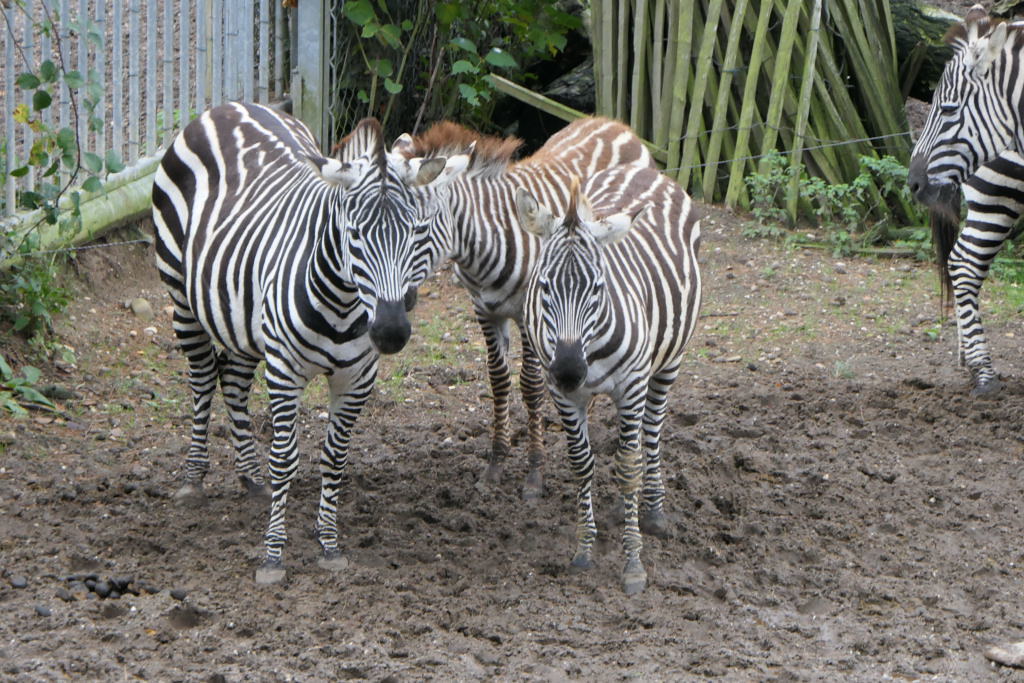The photograph captures a group of zebras within an enclosure, standing on very muddy ground that's dotted with dirt clods, rocks, and zebra feces. Three zebras occupy the center of the frame: two of them facing the camera, and a third partially obscured behind them, sporting distinctive brownish stripes instead of the traditional black. On the far right of the image, two zebras are partially visible; one shows just its head while the other reveals a hind leg and the tail.

The environment around them is cluttered with various fencing types. Towards the left, there is a small wood fence stained green at the bottom, with a large vine hanging down. Overlapping this wood fence is a chain-link and metal gate structure, standing in the upper left corner. In the background, there’s a makeshift fencing made from bamboo posts tied together. Green, brown-stemmed plant growth can be seen sporadically around the enclosure, adding a touch of greenery to the scene. The overall atmosphere is one of contained wilderness, with the muddy ground showing clear signs of the zebras' activity.